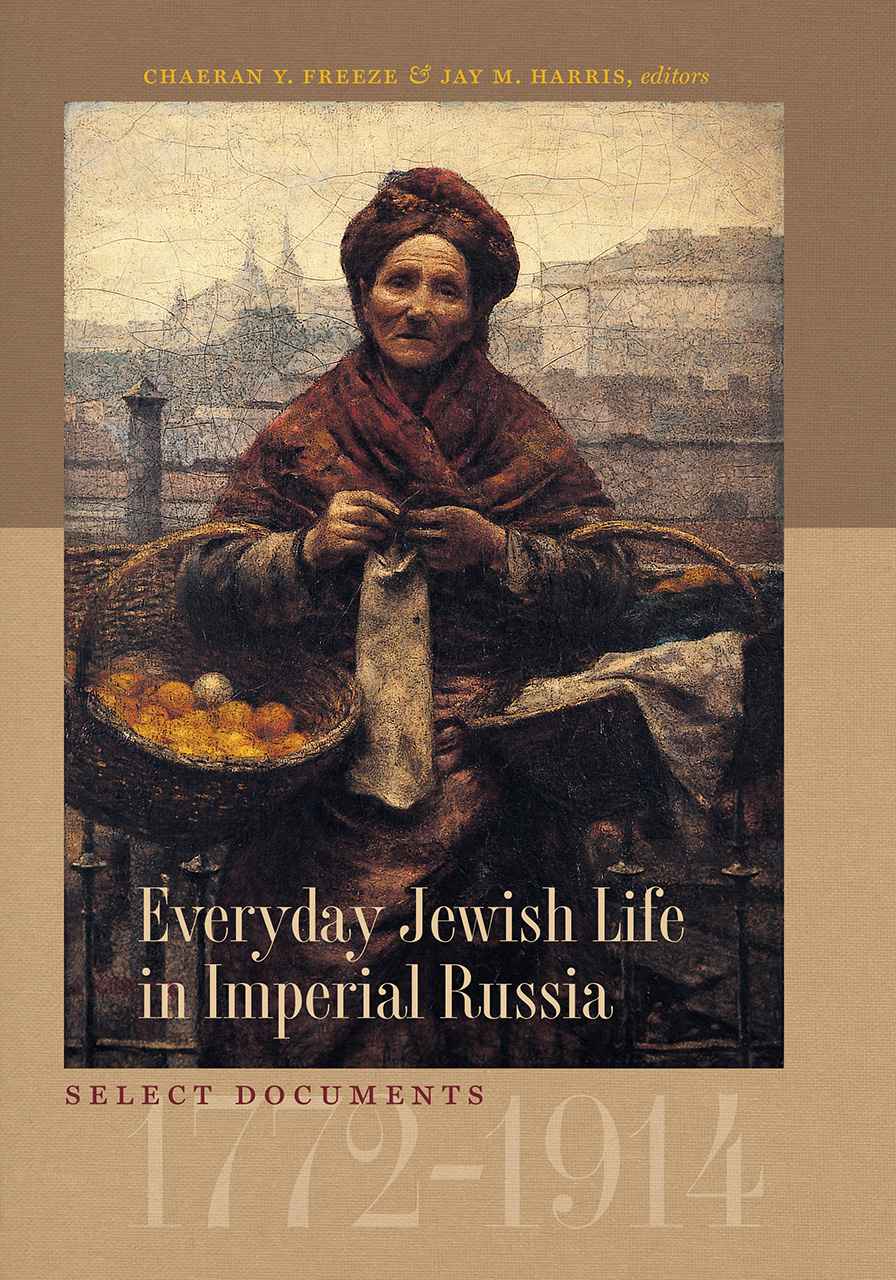The cover of the book, "Everyday Jewish Life in Imperial Russia: Select Documents 1772-1914," edited by Charon Y. Fries and J. M. Harris, features a visually compelling image. It highlights a painting or a photograph of an elderly Jewish woman from Imperial Russia, depicted as a dignified peasant carrying two baskets. The woman appears weathered and hardworking, wearing a brown shawl and a headpiece. The basket on her right has bright orange fruits, possibly oranges, while the left basket, covered partially with cloth, might contain laundry. She stands against a backdrop of an old, possibly cracked cityscape, adding to the historical ambiance of the scene. The cover combines a brownish and tan palette, with the title and subtitles in white and yellow text, respectively. The image powerfully conveys the toil and resilience of Jewish life in the specified era.